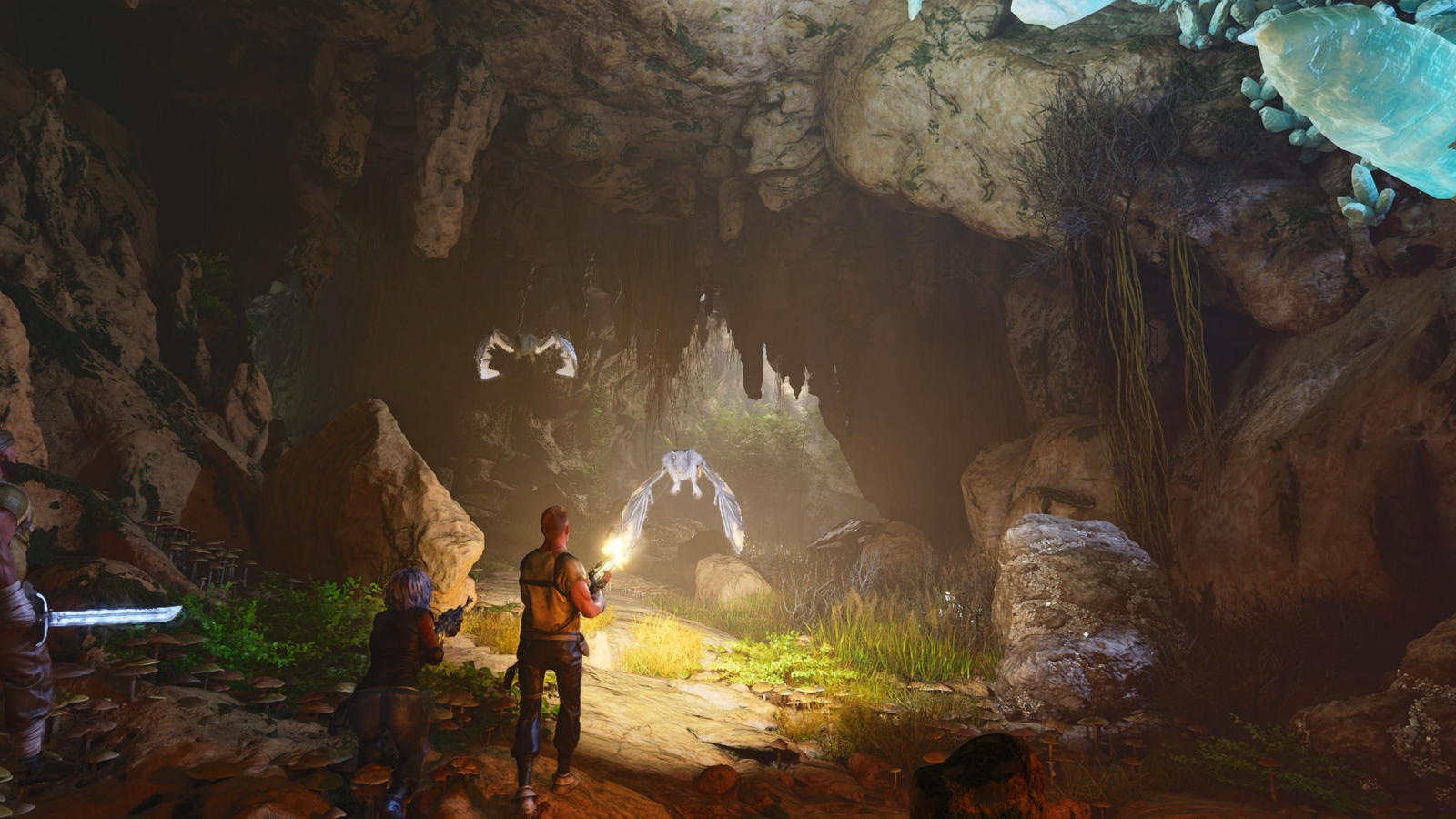The image depicted is a highly detailed computer graphic still frame from a video game, set within the cavernous depths of a cave. The environment is defined by jagged rocks and an array of stone formations, creating a shadowy backdrop illuminated sporadically by turquoise-colored crystals embedded in the cave's ceiling. Central to the composition are two characters, their backs turned to the camera; the one on the left appears to be a woman, while the one on the right seems to be a man. Both are armed with guns and are in the midst of firing at a large, illuminated white creature resembling a bat or bird in the background. Another, smaller winged creature appears near the top left of the image. Trailing the two gun-toting characters is a third individual wielding a long sword, suggesting a team dynamic as they navigate the stony underground expanse. The contrast between the shadowy cave and the glowing creatures and crystals adds a dramatic flair to the scene.